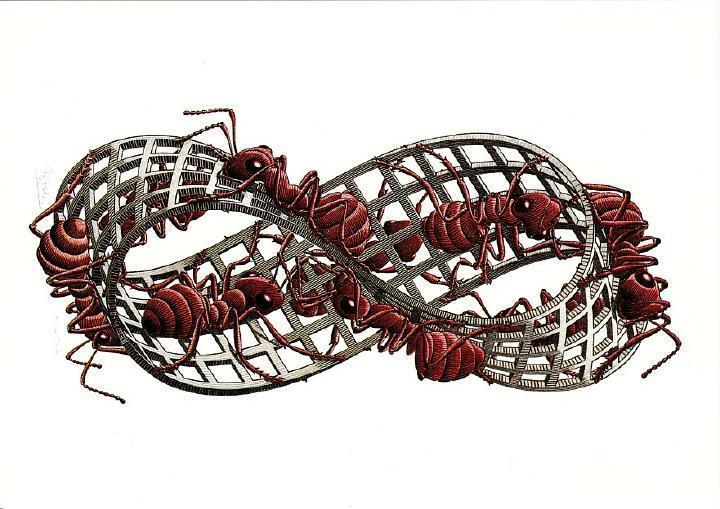The image depicts a close-up, digitally created scene featuring numerous red-brown ants crawling on a silver, wavy metal structure resembling a crisscrossed, twisted figure-eight or infinity loop. The metal has a waffle-like pattern with four squares. The large size of the ants relative to the structure allows for significant detail on their bodies, including twisted ends and intricate textures, suggesting the image is highly zoomed in. The ants are distributed across the metal track, giving an appearance that blends both lifelike and slightly cartoony elements. The scene lacks any text or indication of time, focusing purely on the intriguing interplay between the detailed ants and the intricately designed metal framework.